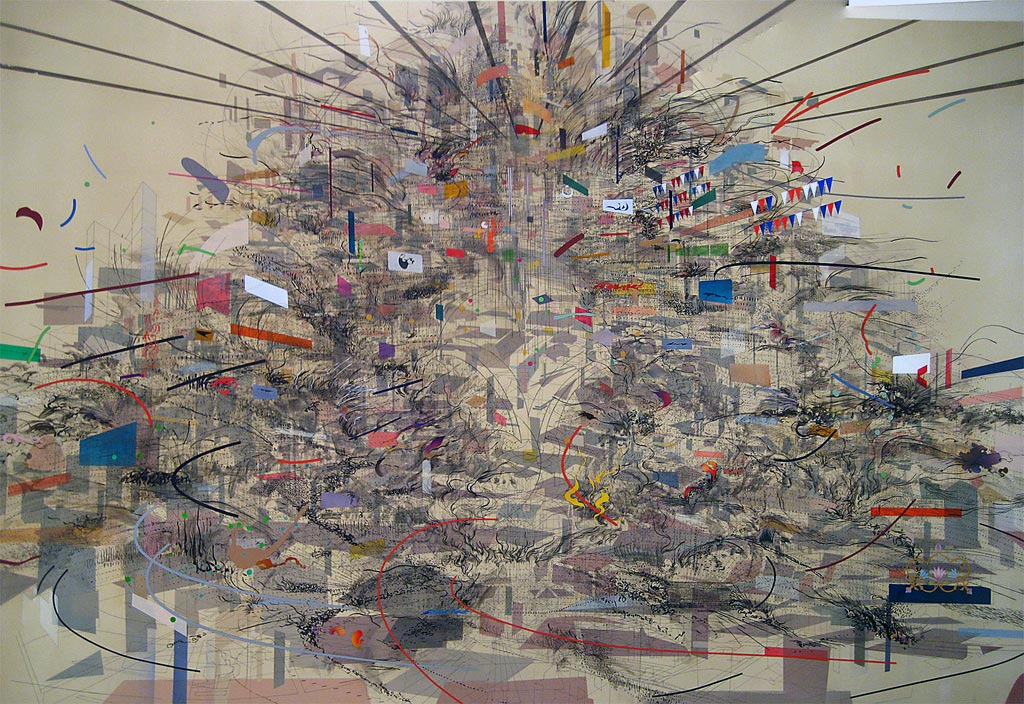This captivating abstract painting, sizable and bursting with energy, features a complex arrangement of chaotic yet intriguing elements that draw the viewer in. The background sets a calming foundation with a light tan hue, against which an array of vibrant details explode in a riot of color and form. Dominating the upper right section are pennant-like flags in red, white, and blue, adding a festive yet cluttered feel. Scattered throughout are diverse shapes—rectangles, squares, and other random forms—rendered in a full spectrum of colors, evoking the randomness of a scattered rainbow. The scene is punctuated with numerous black, squiggly lines and spiky lines emanating in all directions, contributing to the painting's overall sense of dynamic motion and layered complexity. Here and there, you'll notice irregular symbols, red dots, and wavy yellow lines interspersed amid the multicolored blocks and hazy gray patches. Predominantly composed of gray and beige tones interwoven with vivid accents, the artwork feels like a whirlwind of activity—lines and shapes jumbled together yet resonating with a strange, palpable harmony.